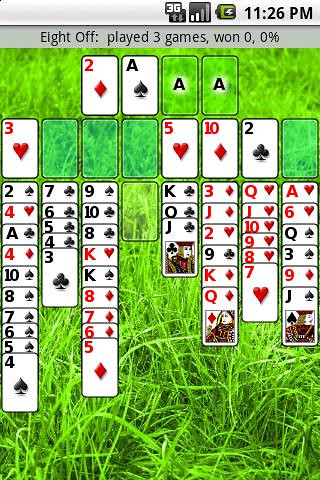This screenshot, taken from an Android device at 11:26 PM, captures a moment in a digital card game. The status bar indicates the phone is fully charged and currently on a 3G network. The game in focus is "8 Off," visibly set against a grassy background. The player has engaged in three games thus far, yet has not secured a win. The interface displays various stacks of cards, with the user strategically navigating through them, pondering their next move in hopes of clinching a victory.